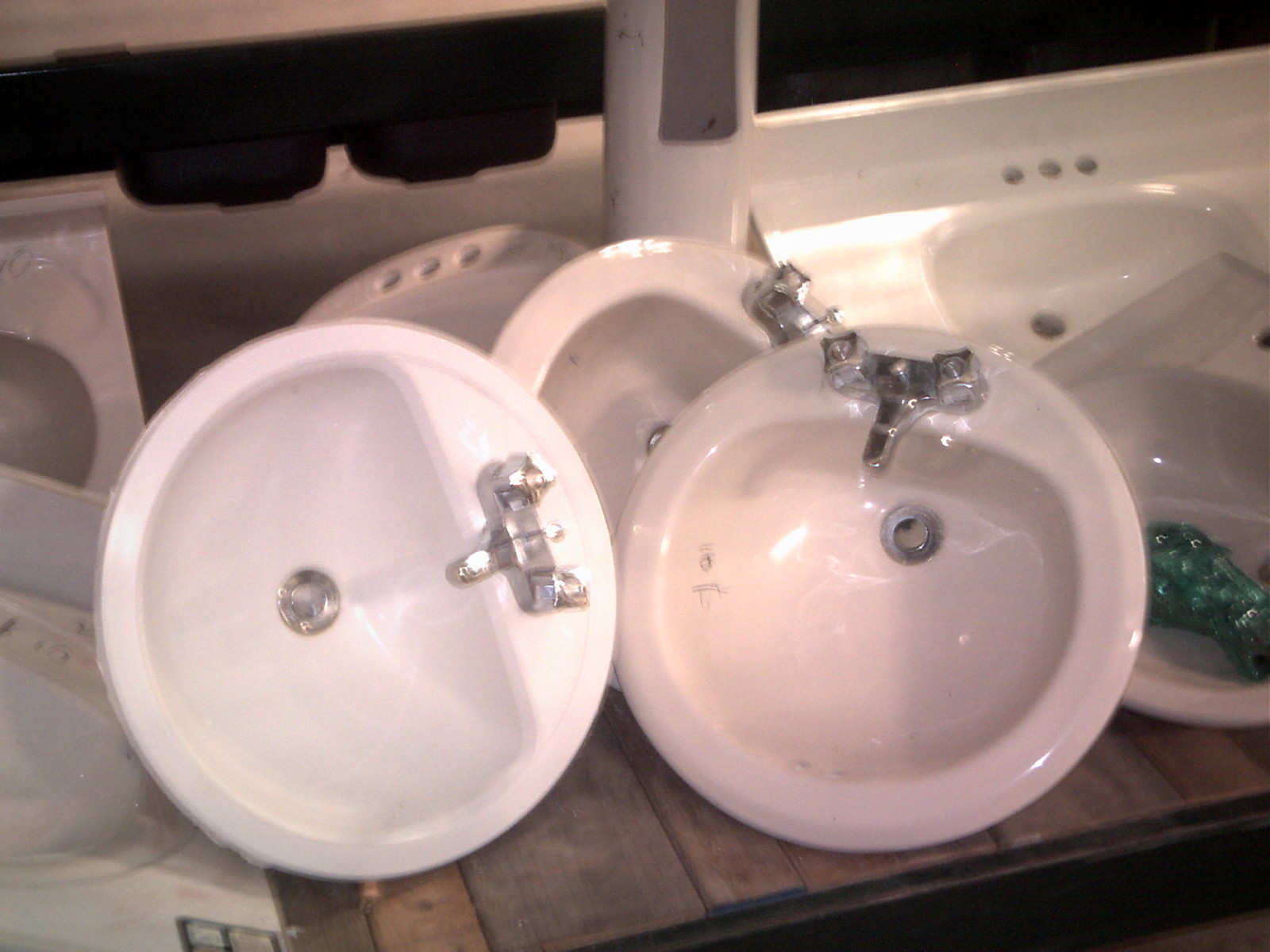The photograph depicts a slightly blurred yet brightly lit indoor scene featuring an arrangement of ceramic sinks typically found in bathrooms or washrooms, all resting on a wooden pallet that is partially visible in the foreground. The sinks vary in shape and size; some are circular or oval, while others in the background have a rectangular form. Their colors range from brilliant white to off-white cream. Notably, some of the sinks have silver mixer taps, plungers, and plugs already installed, while others, particularly those at the back, only have pre-drilled holes for future fittings. Additionally, there are porcelain countertops and vanity tops beside the pallet. One detail that stands out is a green plastic bottle placed inside one of the sinks. The chrome on the fixtures shines with a bright silver hue, adding contrast to the varying whites of the sinks. Despite the soft focus, the image clearly portrays a diverse collection of uninstalled sink basins intended for countertop integration.